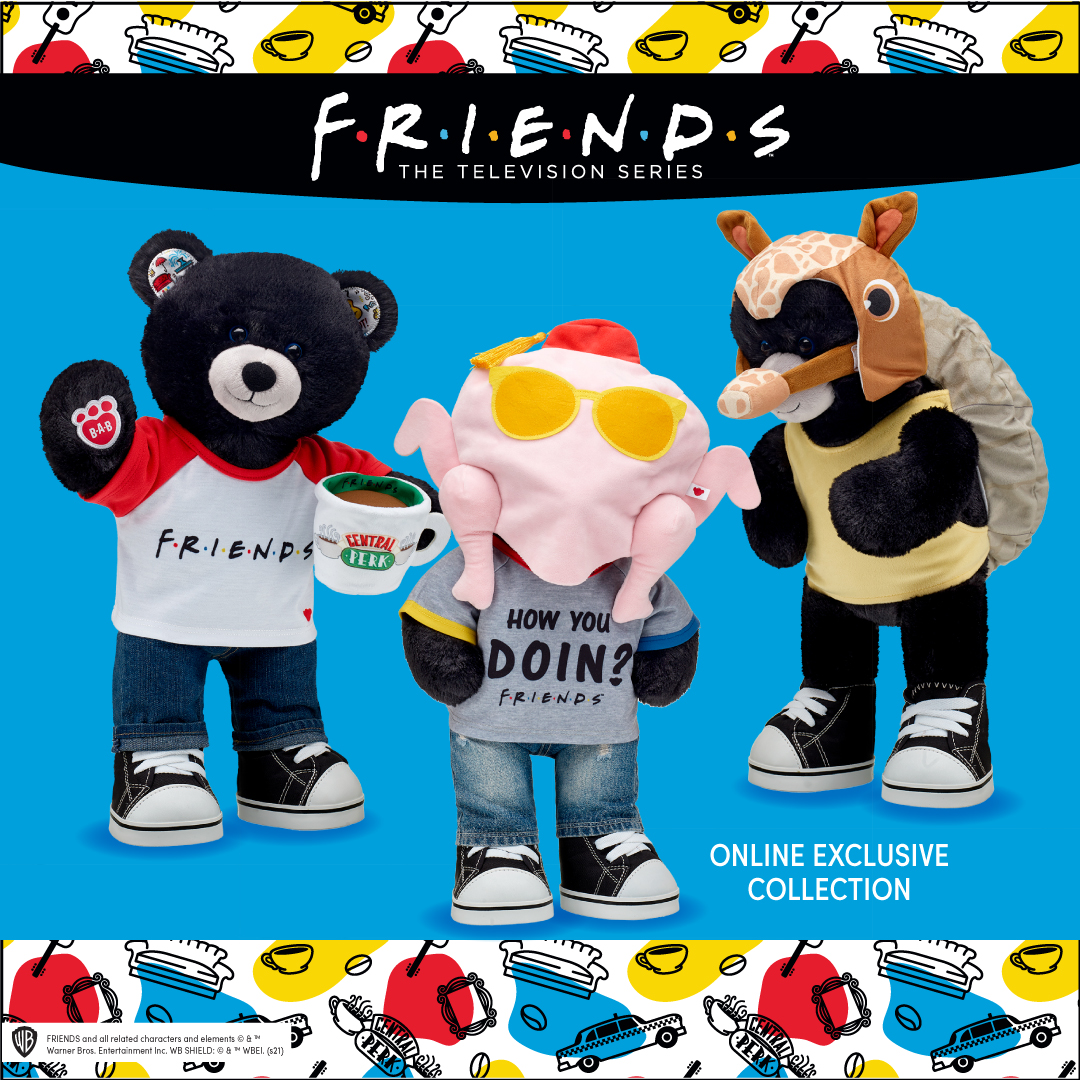The image is an online advertisement for a Friends-themed collection of Build-A-Bear teddy bears, set against a white background. At the top, a banner displays "FRIENDS" in all capital letters with red, blue, and yellow dots between each letter. The three bears, all black, are dressed in outfits inspired by memorable moments from the Friends TV show. The bear on the left wears a white FRIENDS t-shirt with red short sleeves, blue jeans, and black and white Converse sneakers. The central bear is notable for wearing a raw turkey costume on its head, paired with sunglasses, a gray short-sleeved shirt that says, "How you doing?," and light blue jeans. The bear on the right sports a giraffe head helmet and a yellow shirt. The bottom of the image features a pattern showcasing various Friends icons, including Phoebe's taxi, the iconic couch, coffee cups, and the Central Perk logo. In the lower right corner, the image is tagged as an Online Exclusive Collection.